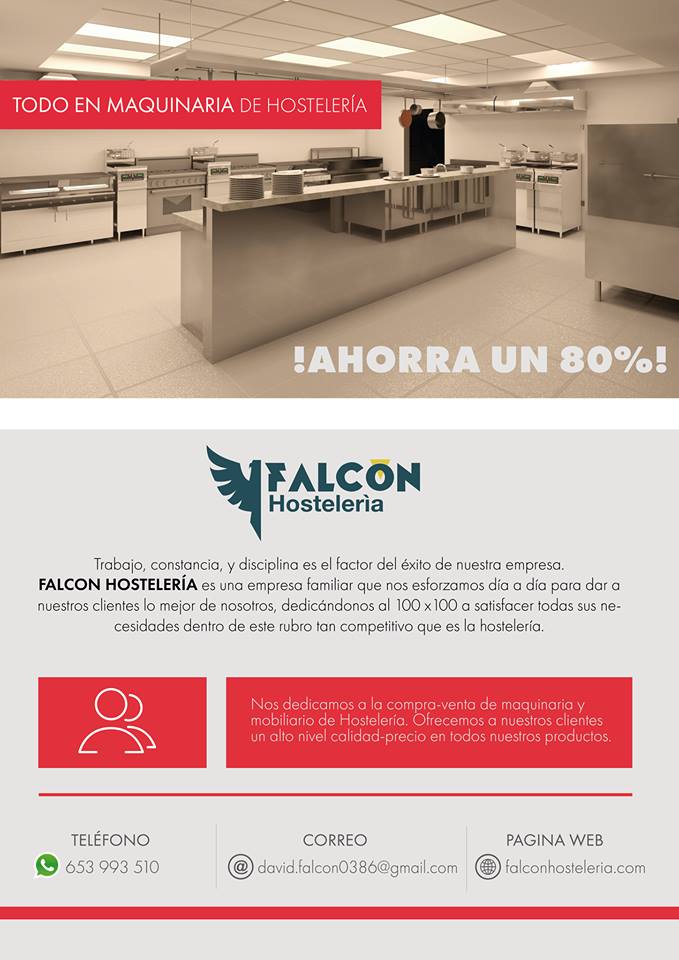The advertisement, written entirely in Spanish, promotes a company named "Falcon Hostelería." It is divided into two sections. The top section features a high-end, modern, industrial kitchen that appears to be for commercial use, such as in a restaurant or business. The kitchen includes multiple stoves—two visible in the foreground and likely two more identified by overhead vent hoods in the background. Hanging pans, stainless steel appliances, and a large center island can also be seen in this empty kitchen setup. A red banner with white lettering is visible on the left side of the image. The bottom section of the advertisement displays the company’s name, "Falcon Hostelería," with a partial image of a falcon in blue. It also provides contact information: a telephone number, an email address, and a website, all centrally located at the bottom of the ad.